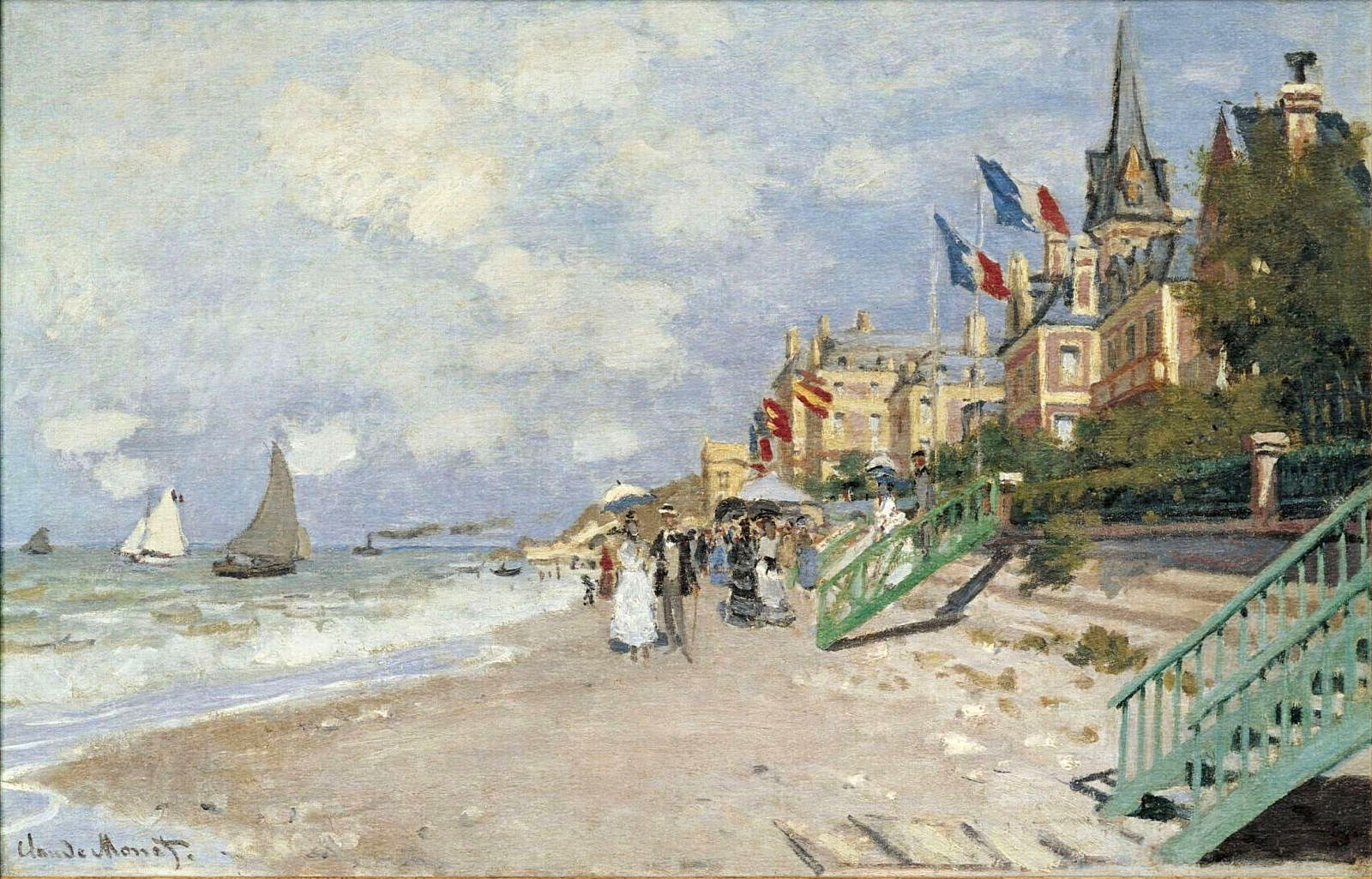This impressionistic painting titled "The Beach at Trouville" by Claude Monet depicts a tranquil beach scene during the day. In the foreground, the sandy shore meets the blue ocean water, with white foam and lavender-tinted pools lapping against the coastline. Sailboats with both brown and white sails, as well as a steamship emitting plumes of steam, can be seen on the water. The background reveals a vast sky painted in shades of blue and purplish violet, adorned with numerous white, puffy clouds.

On the beach, the scene is lively with people strolling along the shore, all dressed in formal attire. Prominently, a woman in a white dress holding a white umbrella walks beside a man wearing a black jacket and gray pants, holding a cane. Nearby, another couple is spotted, with one wearing a straw hat. To the right, two women walk away from the couples, one in a black dress and the other in a gray dress with a black belt. Another notable figure is a woman in a red dress, also holding an umbrella.

To the right-hand side of the image, a green-banistered stairway leads up to a boardwalk lined with buildings adorned with French flags in blue, white, and red stripes. Among these structures, one stands out with a tall spire, resembling a church. These buildings, with their varied architectures, including some brick constructions with man-sized roofs and a gable roof section, add depth to the composition. This masterpiece not only captures the essence of a leisurely day at the beach but also showcases Monet's signature impressionistic style.